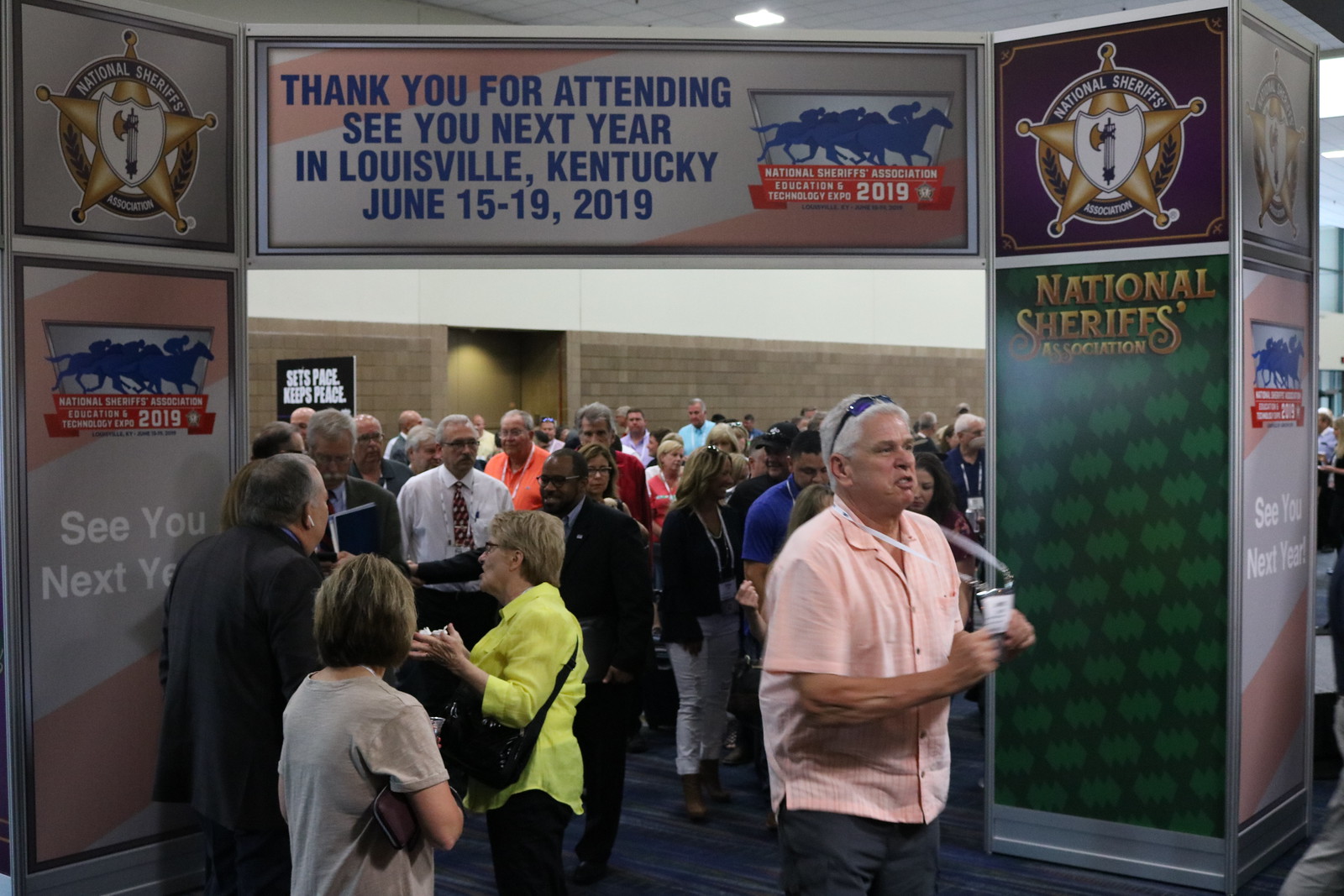This photo captures the bustling scene at the backside of an archway made of posters inside a convention hall. The archway, adorned with text and images including a sheriff's badge, prominently displays the message: "National Sheriffs Association. Thank you for attending. See you next year in Louisville, Kentucky, June 15 to 19, 2019. National Sheriffs Association Education and Technology Expo, 2019." Beneath the archway, a crowd of older attendees, mingling and conversing, begins to make their way through. Closest to the camera is an older man with gray hair, wearing a peach short-sleeved shirt and sunglasses perched on his head. He holds his lanyard badge out in front of him, appearing to shake it and yell, adding to the lively atmosphere of the event.